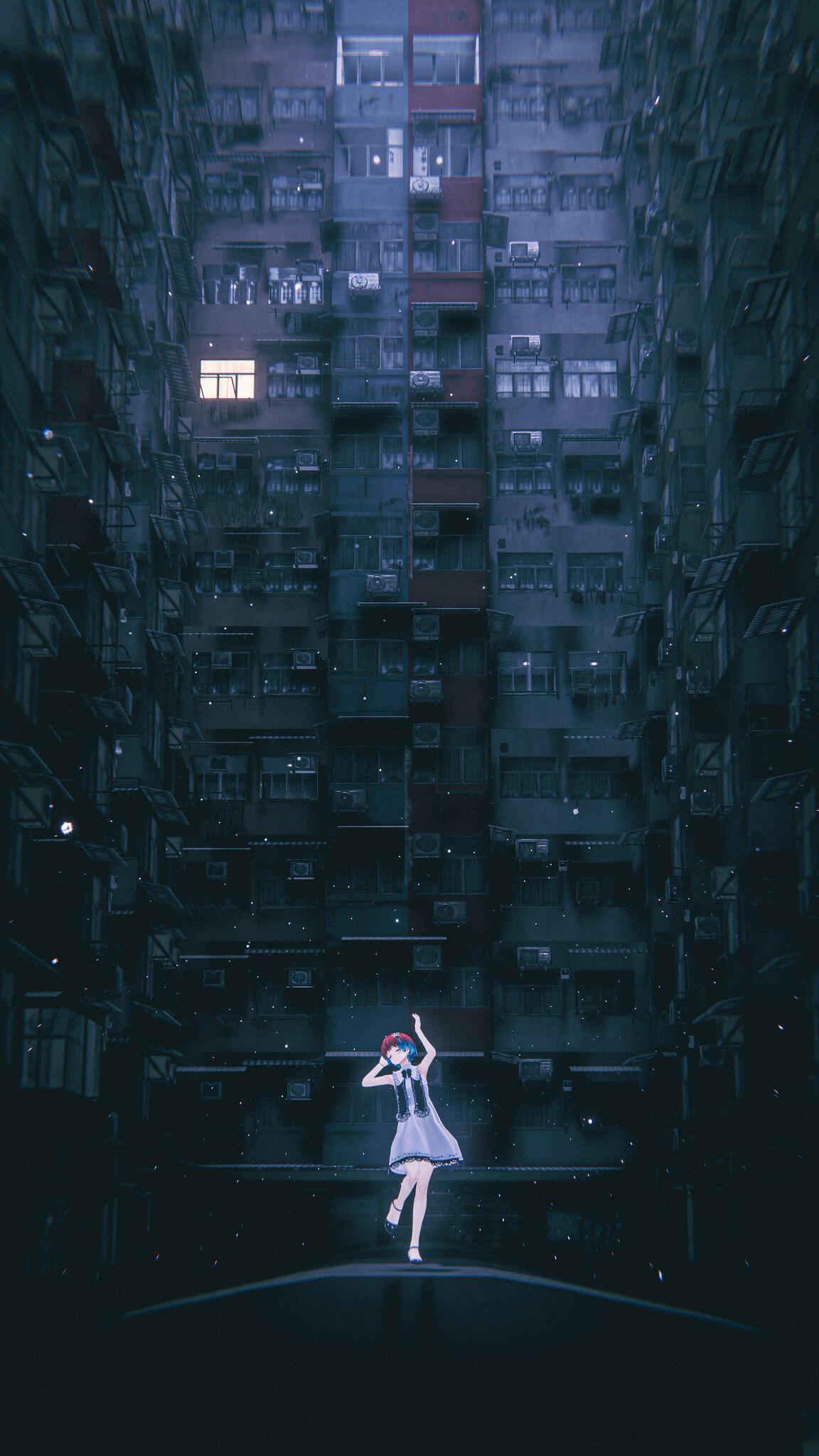The image depicts a digital screenshot from an anime featuring a luminous female character, almost resembling a hologram, positioned in a dark alleyway against the backdrop of a towering, skyscraper-like apartment complex. The scene is shrouded in darkness, with only one window in the vast array of apartments brightly illuminated, hinting at the presence of life within the otherwise dim building. The anime character, a petite girl with striking blue hair, is dressed in a small, sleeveless dress and red beret, complemented by slip-on shoes. She appears to be dancing, with one hand over her ear and the other raised in the air, her body curved elegantly to the right. The detailed composition underscores the contrast between the brightly lit character and the dark, expansive urban environment behind her.